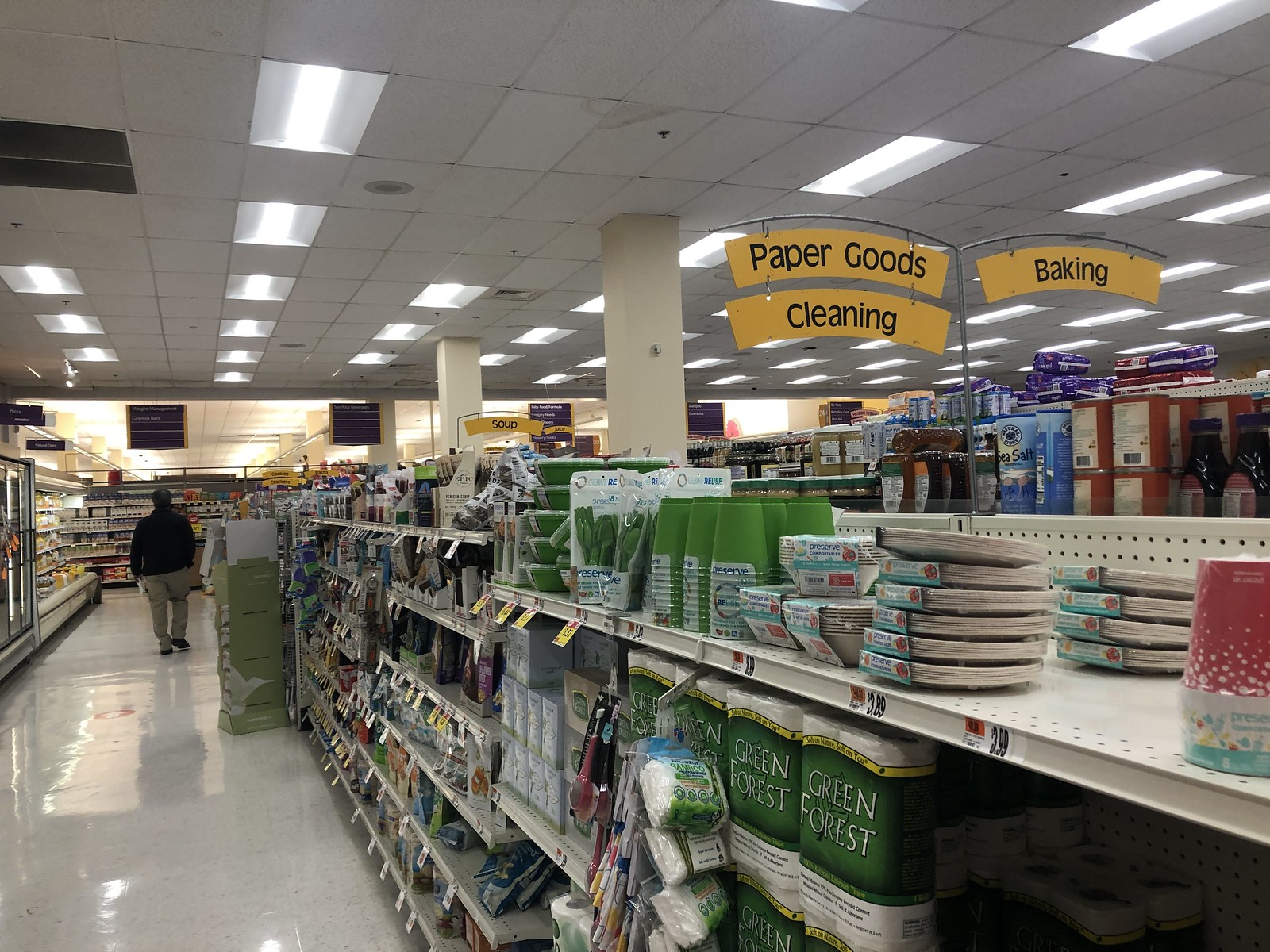The image captures the interior of a retail store aisle lined with metal shelving. The aisle, meticulously maintained with highly waxed vinyl tile flooring, features a variety of paper goods and cleaning materials. Metal shelves of uniform width, but varying heights, extend from the lower right-hand side towards the left center of the frame. A customer, a slightly overweight gentleman in a dark-colored coat and light-colored pants, is walking down the aisle on the left side. His dark hair is visible as he meanders through the store.

White, large, rectangular columns support the ceiling, which consists of a drop-down white tile design with fluorescent light fixtures embedded within. Signage is displayed on small metal stands, with category markers embedded in slightly arched yellow rectangles with black lettering. The current aisle is labeled for paper goods and cleaning supplies, while the adjacent aisle is designated for baking goods.

On the upper shelves, a selection of paper plates and plastic cups is visible, while the shelf below features green-hued paper towels, likely from the Green Forest brand. The meticulous organization and cleanliness of the aisle provide a welcoming shopping environment.